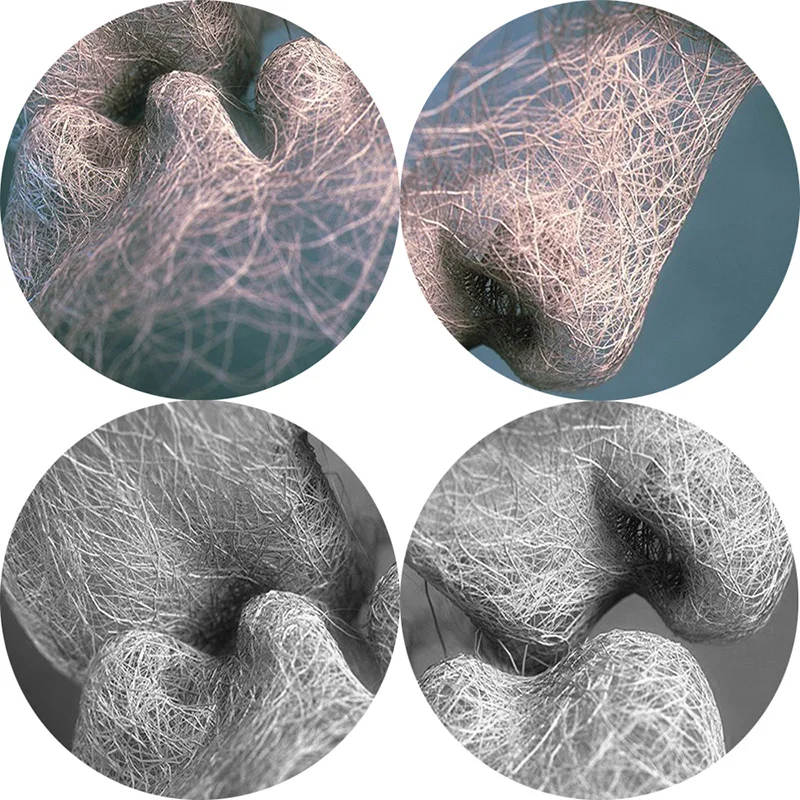The image depicts four circular close-up sections of a highly detailed, sculptural art piece made of interwoven, fibrous materials that resemble white thread or bristles. These circles are arranged in a 2x2 grid against a plain white background. The top two circles feature a light blue background, while the bottom two have a grey background. 

- **Top Left Circle:** Shows a textured, fibrous area that suggests the contours of lips touching a chin or perhaps two faces meeting, though the exact shapes are rather abstract and difficult to discern clearly.
- **Top Right Circle:** Clearly displays a human nose made from dense and less dense portions of the thread-like material, showing the characteristic slant and shape of a nostril.
- **Bottom Left Circle:** Contains shapes reminiscent of lips and a chin, possibly depicting two faces in close proximity or kissing.
- **Bottom Right Circle:** Appears to show a partial face with a nose and nostrils, and an edge that resembles lips, indicative of two faces kissing.

These intricate sculptures exhibit a unique texture and depth, capturing facial features in a semi-abstract manner using the intricate interplay of the fibrous material.